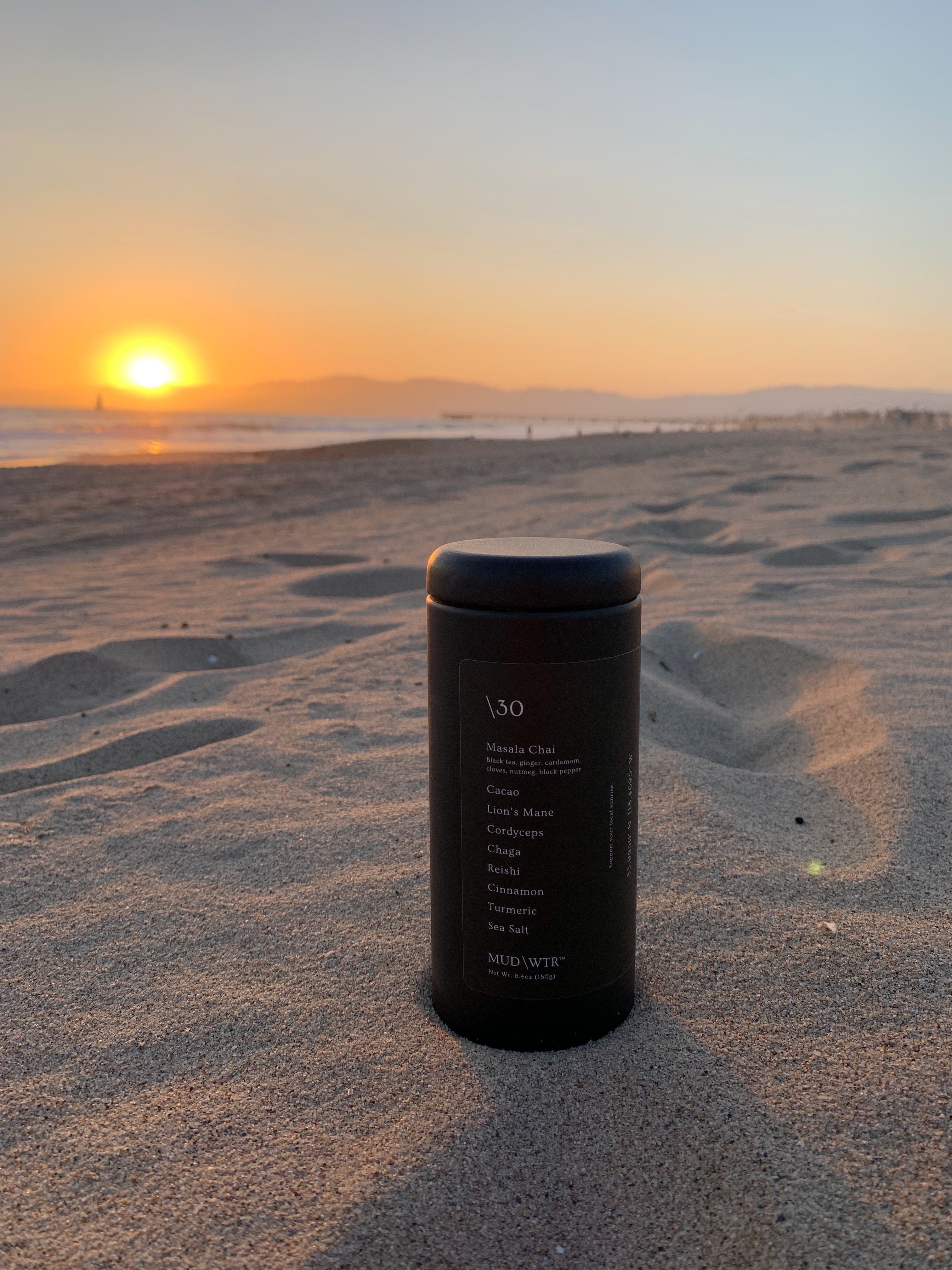The image depicts a black canister labeled "Mud/Wtr" sitting in the sand on a beach during either sunrise or sunset. The long, cylindrical canister features a small cap and bears white lettering that lists ingredients such as masala chai, cacao, lion's mane, cordyceps, chaga, reishi, cinnamon, turmeric, and sea salt, with the number 30 prominently displayed. Surrounding the canister is a sandy beach marked by footprints, with the ocean visible in the distance. Silhouetted figures walk along the shoreline, and an island with an indistinct outline of what might be a lighthouse can be seen across the water. The overall atmosphere is calm and picturesque, with no signs of rain, capturing a serene moment at the beach.